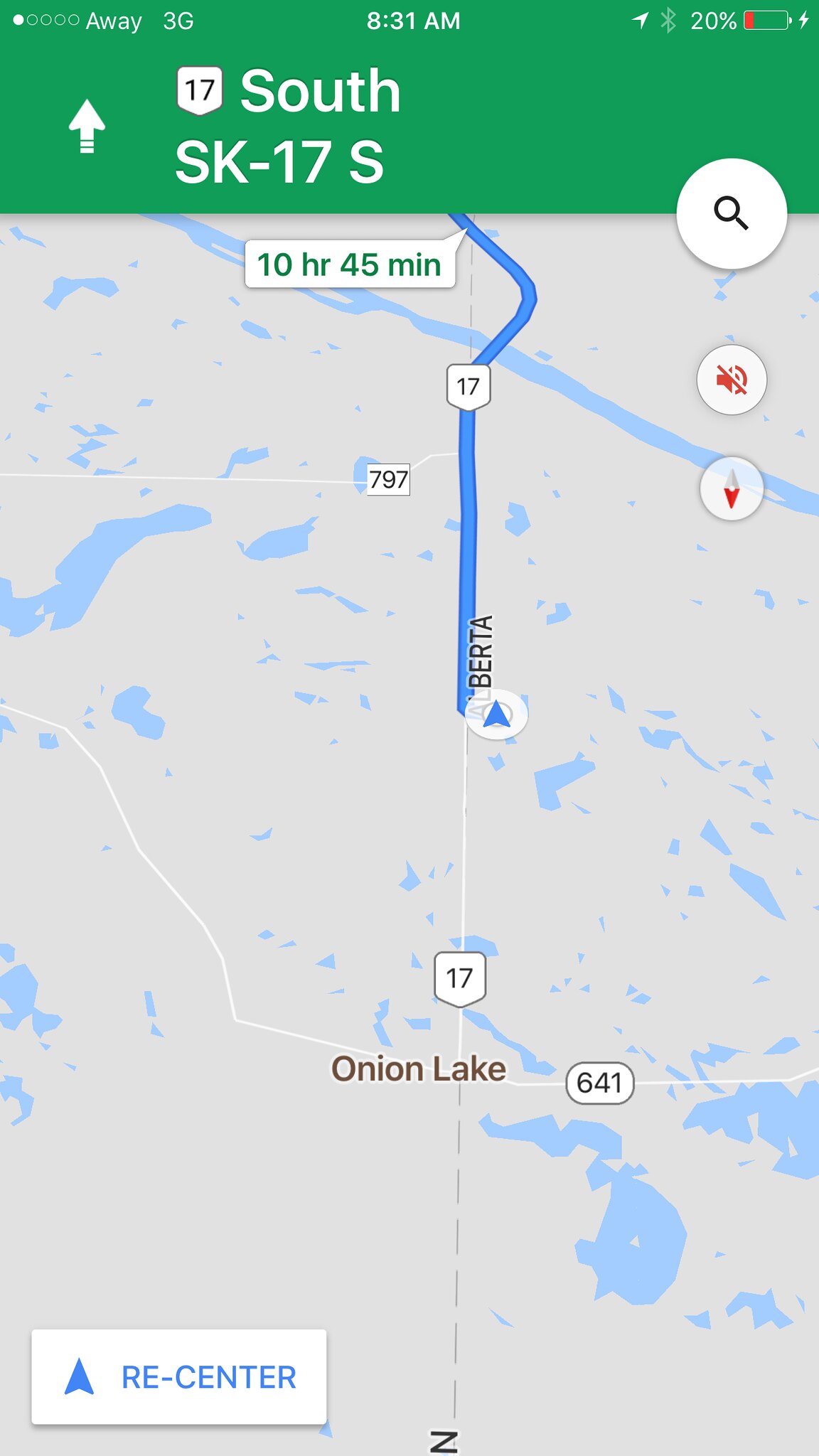This is a detailed screenshot of a Google Maps navigation screen taken on a mobile phone, likely an iPhone. The map prominently displays Highway 17 South (SK-17S) and indicates a navigation route with a remaining travel time of 10 hours and 45 minutes. The starting point and destination are visible, though not specified. The map highlights important locations like Bertha and Onion Lake, and a crossroad marked as 641. The phone screen shows essential data, including a battery level at 20%, a 3G signal with one bar, and the time at 8:31 AM. Additionally, there's a search icon represented by a magnifying glass, and a re-center button at the bottom of the map displayed in a rectangular box. Distinctive features like dark navigation arrows guide the path. The screenshot includes subtle geographic details such as small lakes dispersed across the map.